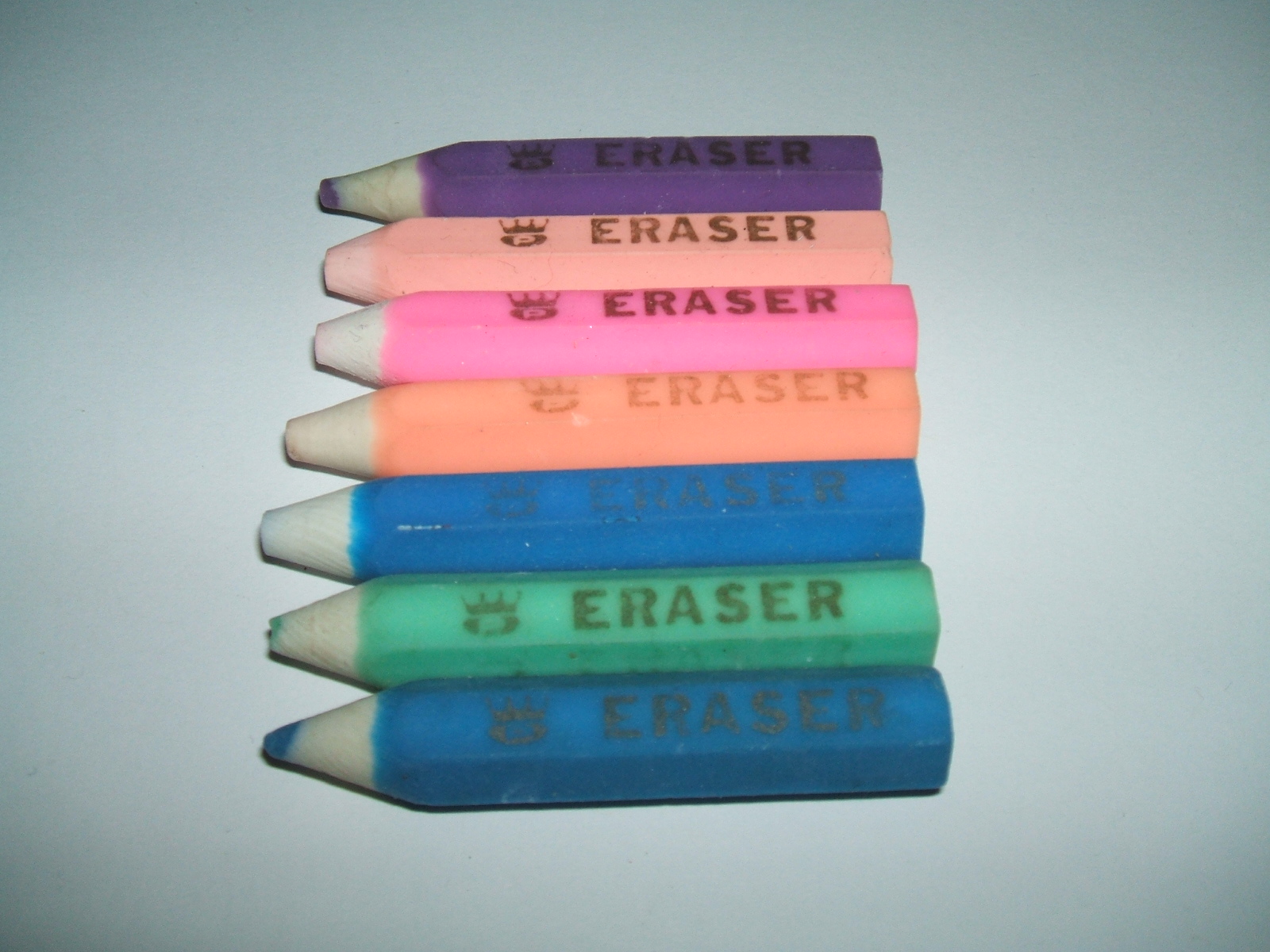The image features seven eraser pens designed to resemble pencil crayons, meticulously arranged horizontally atop a white table surface. Each eraser pen is aligned in a column with their tips pointed to the left and their ends to the right. The colors of these erasers progress from the bottom to the top as follows: dark blue, green, dark blue, orange, bright pink, light pink, and darkish purple. Each pen displays the word "ERASER" in black capital letters along with a logo showcasing a crown and the letter "P" on a black background. The tips, crafted to mimic actual pencil leads, are light brown, with the dark blue eraser at the bottom revealing a visible pencil-like lead, while the others predominantly show the white simulated pencil body, with the exception of the purple one at the top, which again showcases a white tip and a hint of purple. The photograph is imbued with a light bluish gradient hue, adding a subtle overall ambiance to the composition.